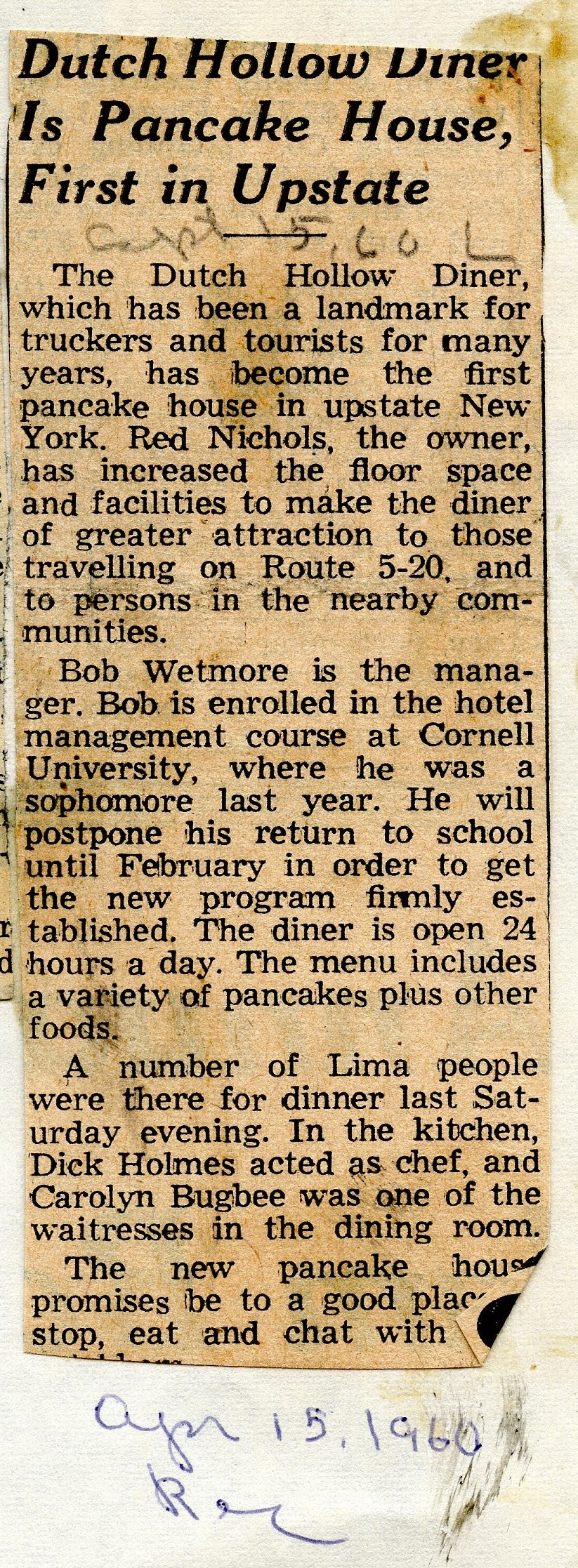The image depicts a color digital scan of an old newspaper clipping, noticeably yellowed with age, and affixed to a slightly discolored, dirty white sheet of paper. In the top right corner of this sheet, there are visible stains and indecipherable pencil markings. The headline in bold black text reads, "Dutch Hollow Diner is Pancake House, first in upstate." The article details that the Dutch Hollow Diner, a landmark for truckers and tourists along Route 520 for many years, has transitioned into the first Pancake House in upstate New York. The owner, Red Nichols, has expanded the diner’s floor space and facilities to attract more travelers and local community members. Bob Wetmore, the manager, is enrolled in a hotel management course at Cornell University and is postponing his return to school until February to establish the new program. The diner is open 24 hours a day, offering a variety of pancakes and other foods. Last Saturday evening, a number of Lima residents dined there. In the kitchen, Dick Holmes served as the chef, and Carolyn Bugbee was one of the waitresses. The article suggests that the new Pancake House will be a great spot to dine and socialize but ends abruptly due to the corner of the paper being folded over. At the bottom, written in blue pen, is the date "April 15, 1960," along with some initials.